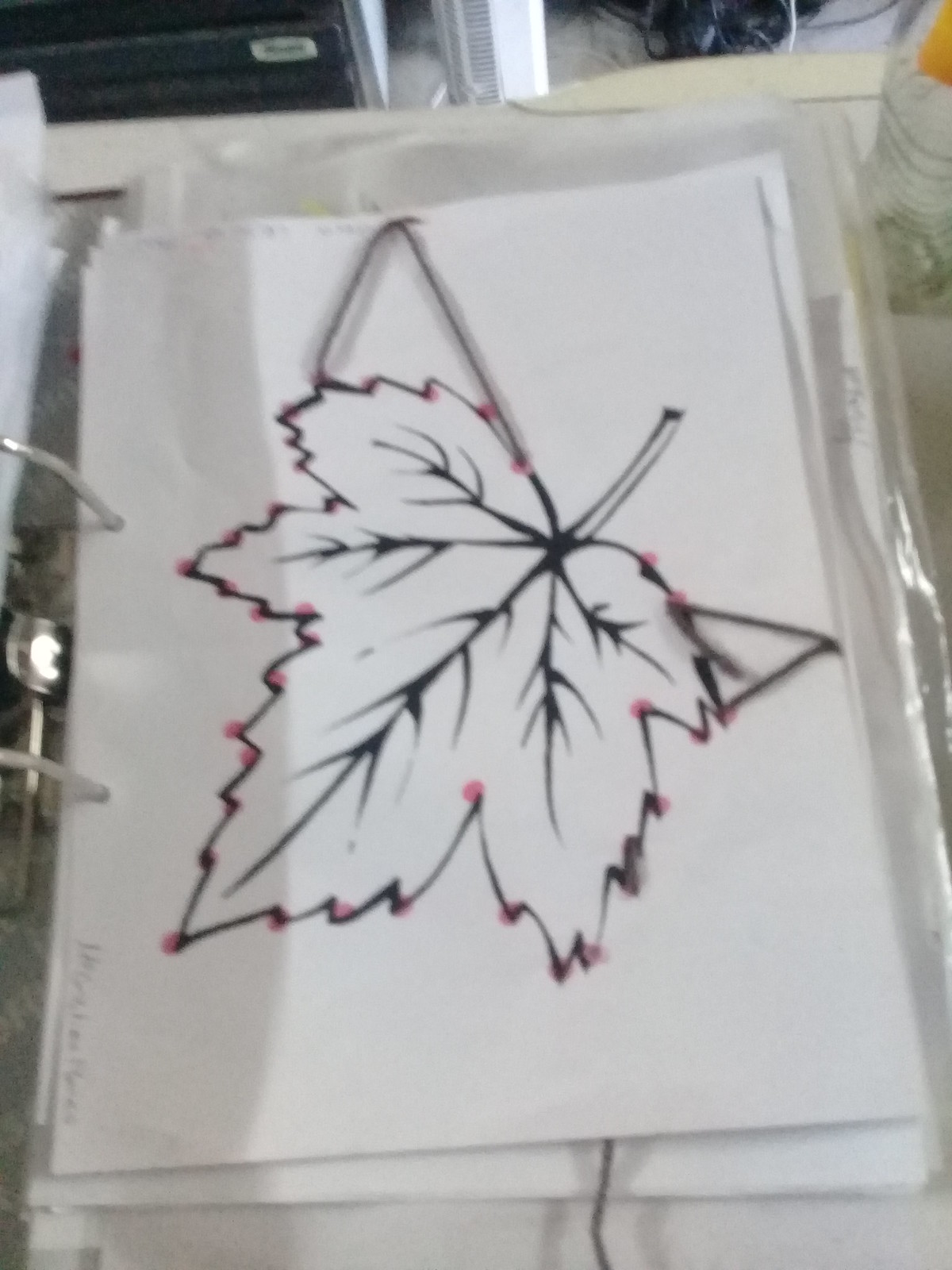A detailed photograph captures a sketch on a crisp, white sheet of paper securely held within a large binder. The left side of the image prominently shows the immense spirals of the binder's spine, designed to be opened by hand for easy paper removal and re-insertion. These metallic spirals are both round and robust, emphasizing the binder's substantial size. The sketch itself features an intricately outlined black leaf, adorned with a series of pink dots meticulously placed along the edges. The leaf's stem is also rendered in black and points towards the top right corner of the photo, positioning the leaf upside down with its tip facing the bottom left. Subtle smudges, likely from either paint or charcoal pencil, blur the area around the right edge of the leaf, adding a touch of artistic imperfection. In the bottom left corner of the paper, a name is delicately inscribed in pencil, oriented vertically to complete this visually engaging composition.